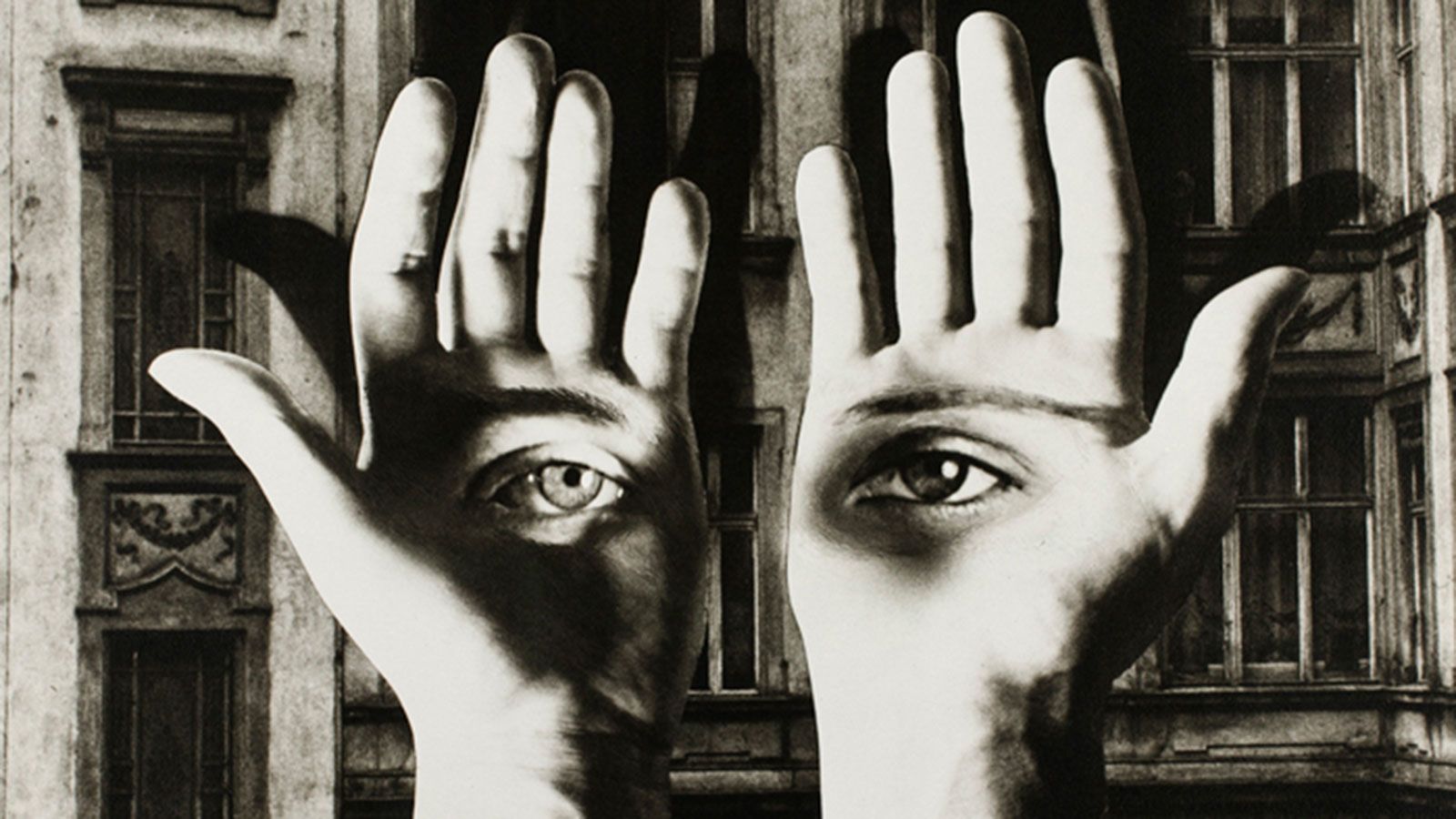The image appears to be a meticulously crafted digital artwork, presented in striking black and white. It features a close-up view dominated by the grayscale silhouette of an old building in the background, revealing intricate window encasements. Prominently in the foreground, two hands are raised, positioned closer to the viewer's line of sight. These hands cast shadows created by a directed light source, which accentuates the contours and natural bends of the thumbs and fingers. Uniquely, each hand has an eyeball set in the palm, framed by surreal eyebrows. These eyes, seemingly of different colors—one resembling brown and the other blue—intently gaze out, establishing an eerie connection with the viewer.